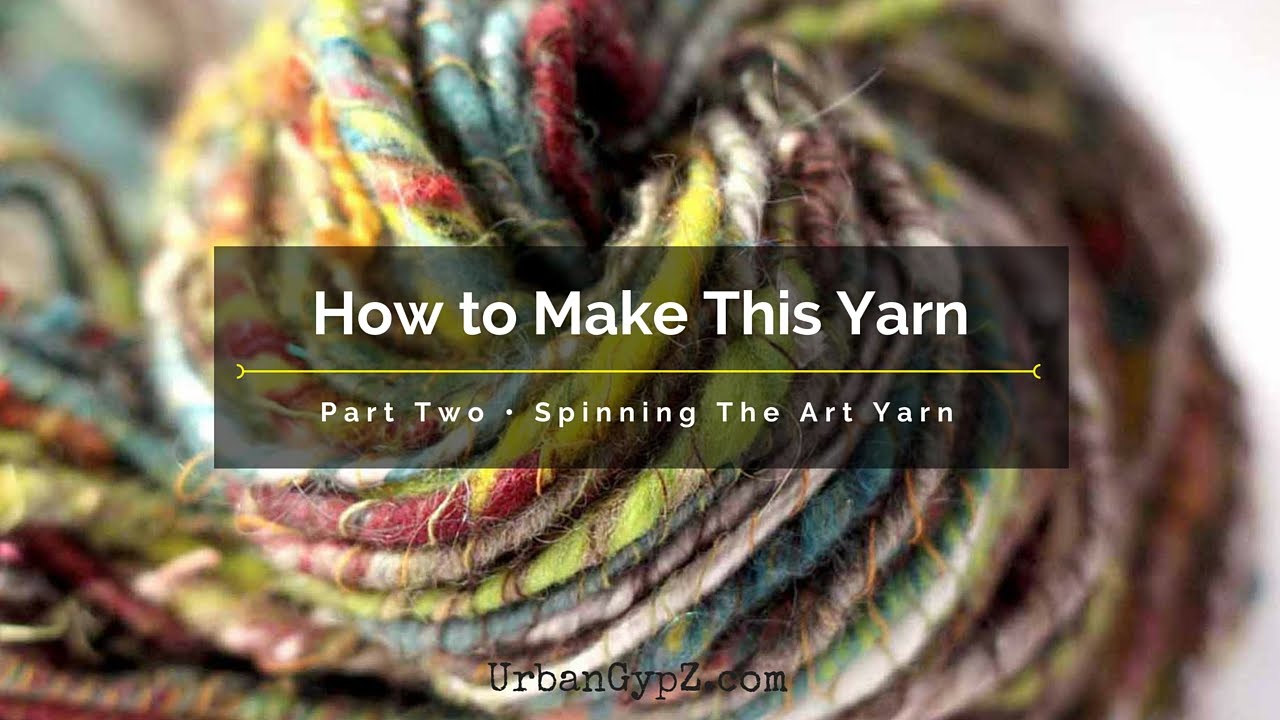This detailed caption describes an image that appears to be either a book cover or a marketing thumbnail for a blog or video on Pinterest. The main focus of the rectangular photograph is a close-up of multicolored yarn, featuring vibrant shades of yellow, red, green, blue, purple, orange, and more, intricately intertwined and knotted together. The colorful yarn is shown against a blurred background, emphasizing its texture and vivid hues.

Over the yarn, there is a slightly translucent black banner with white text. The main title on the banner reads "How to Make This Yarn." Below this, separated by a thin yellow line, it says "Part 2: Spinning the Art Yarn." Towards the bottom of the image, darker black text displays a web address: "urbanGypz.com."